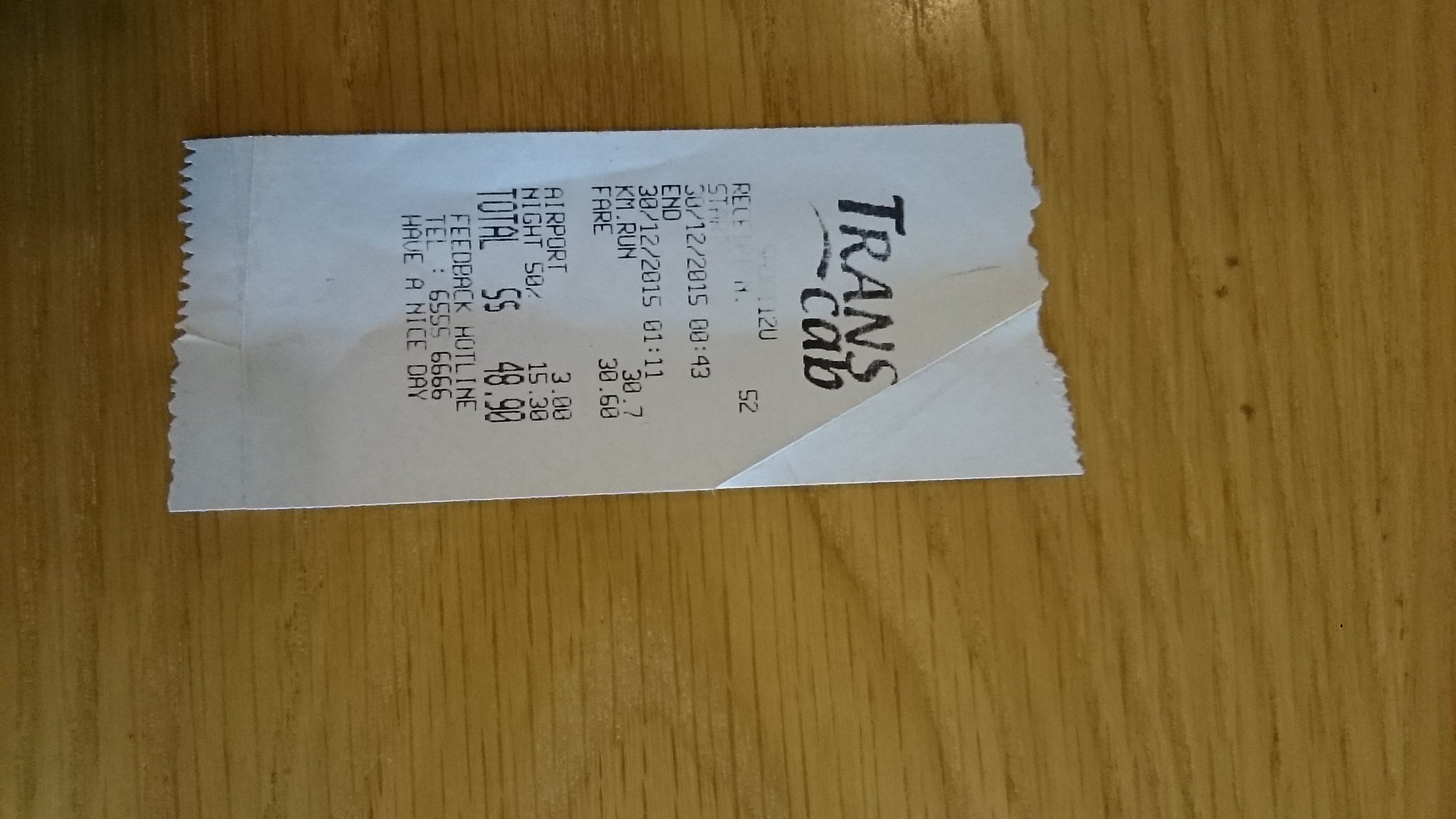The image features a white receipt laying sideways on a light-colored oak wooden floor. The receipt displays the header "Trans Cab" in black text at the top. Below the header, there is some faded information also in black. A date is visible: 12/2015. The receipt details an airport charge of $3 and a total amount of $48.99. Additional text includes a feedback hotline with the telephone number 6555-6666 and the friendly message "Have a nice day" in black text towards the bottom. The receipt has ragged edges at the top and bottom, while the sides are smooth. In the image, the top of the receipt is oriented to the right.